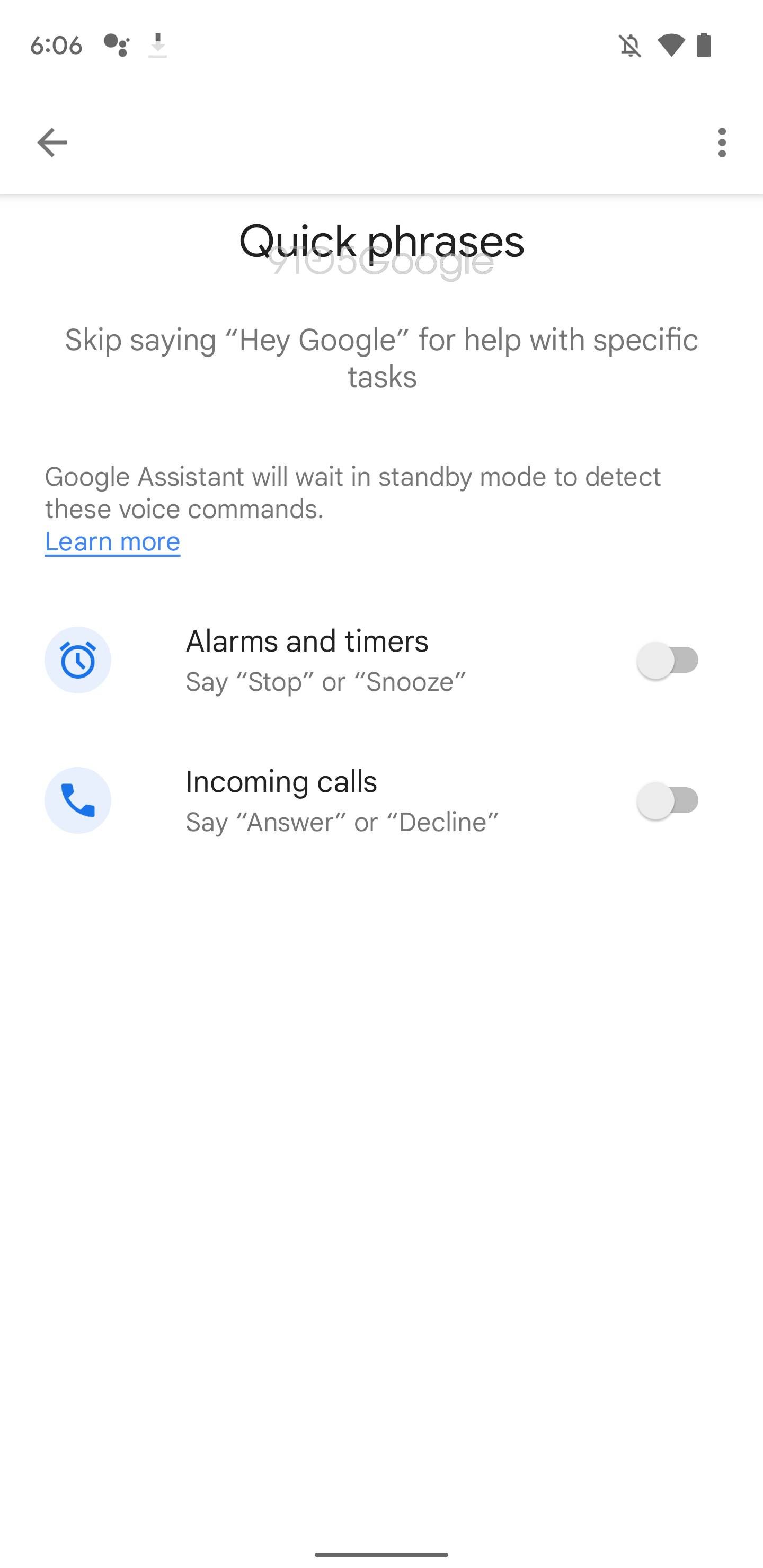Detailed Caption:
The image depicts a smartphone screen featuring the Google Assistant interface. At the top right of the screen, there is a status bar displaying a bell icon, a slash through it indicating notifications are muted, a full Wi-Fi signal icon, a fully charged battery icon, and a left arrow. There are also ellipses representing additional options or menu items. Below the status bar, the interface shows a section titled "Quick Phrases" with options to perform tasks using commands to Google Assistant. 

Highlighted text instructs users to say, "Hey Google," to initiate assistance for specific tasks. A message beneath reads, "Google Assistant will wait in standby mode to detect these voice commands. Learn more." There is also a section dedicated to setting clock alarms and timers, indicating users can say "stop" or "snooze" to control them. 

Further down, a section labeled "Incoming Calls" instructs users to answer or decline calls by speaking the respective commands. The background of the screen is predominantly white, with well-organized text and icons for easy navigation. At the very bottom of the screen, there is a dark icon, possibly representing additional options or settings for the Google Assistant.

Note: The overall layout is clean and functional, aiming to streamline user interaction through voice commands.